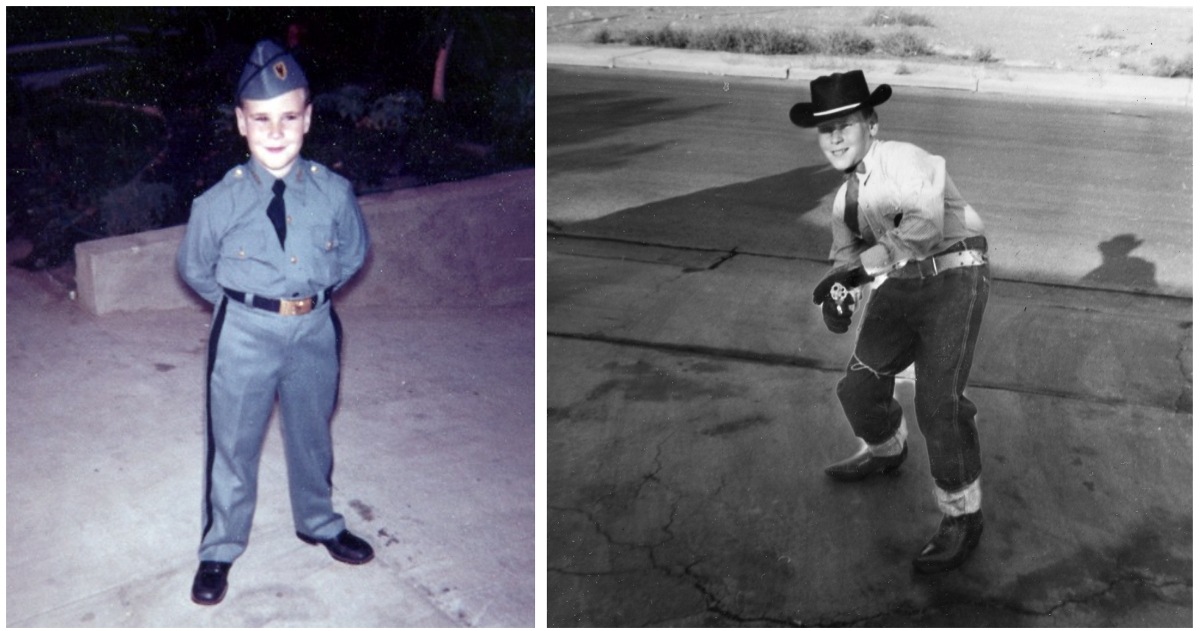The image is a combination of two smaller photographs, one on the left and one on the right, each featuring a young boy dressed in distinctive outfits. 

The photograph on the left depicts a young boy in a gray uniform consisting of a jacket, shirt, pants with black stripes on the sides, black tie, and black shoes. He is also wearing what looks like an army or police cap and has his hands behind his back. The boy stands on a white, dull, paved pathway with a dark indistinct background, giving the impression of a dated photograph despite being in color and slightly blurry.

The photograph on the right is in black and white and shows another young boy wearing a white button-down shirt, dark pants, and dark shoes. He is adorned with a black cowboy hat and black gloves, holding what appears to be a replica revolver in his hands. The boy is smiling and stands with his feet apart and both hands on the fake revolver. The background shows a sidewalk and a paved road with another light-colored stone sidewalk further back, providing a clear outdoor setting.